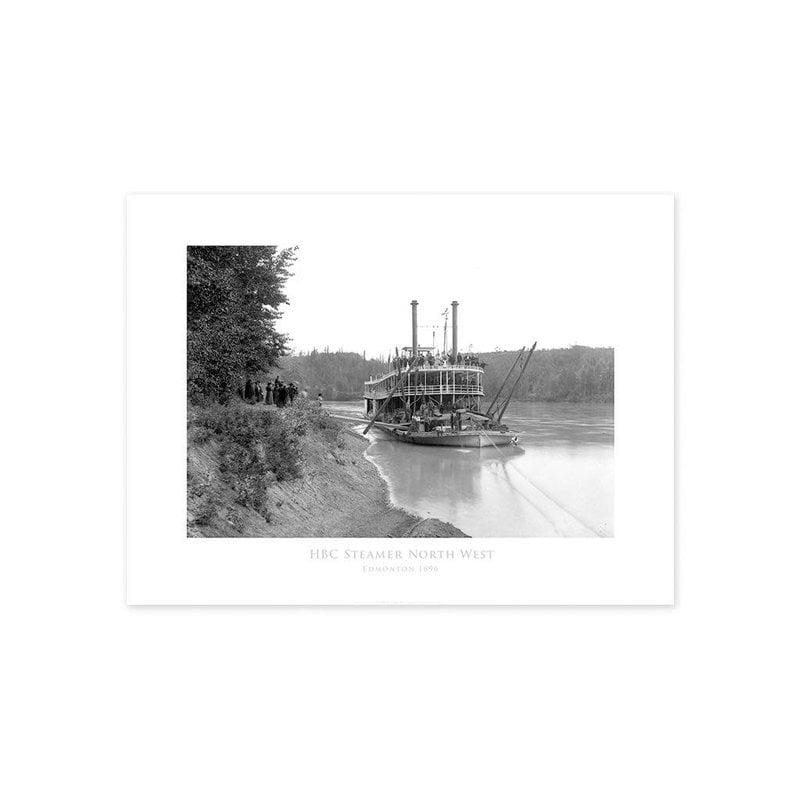The black-and-white photograph, titled "HBC Steamer Northwest," captures an evocative scene from a bygone era. The centerpiece of the image is a large steamboat, anchored in a relatively shallow, medium-sized river near the shore. The boat, adorned with white railings on its second tier and tall pillars on top, exudes a sense of grandeur, hinting at its once-prominent role in river transport. Despite the historical photograph being somewhat grainy, a crowd of people dressed in period-specific black clothing can be seen standing to the left of the boat, seemingly preparing to board via a ramp leading from the riverbank to the vessel. In the background, distant trees, and possibly a mountain, complete the picturesque scene, enhancing the timeless quality of the image. The wide white border and the cardstock framing of the photograph further emphasize its age, giving it an authentic, antique feel.